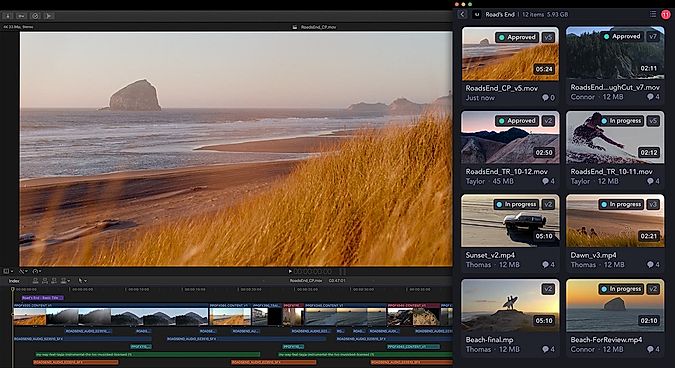The image depicts a web page that appears to be a video editing or approval platform. The main section of the page displays a beach scene featuring dried grass, a large rock in the water, sandy shores with tire tracks, and the main video file named "roadendcpb5.move," which has just been approved. 

On the right-hand side of the page, there is a series of thumbnails arranged vertically, each associated with timestamps and various approval statuses. These thumbnails include:
1. An image of mountains with trees labeled "roadsendungcutv7.move," approved.
2. Another mountain image named "roadendtr1012.move," also approved.
3. A snapshot showing a person waterskiing identified as "roadendtr10-11.move," currently in progress (v5).

Additionally, there are video files with specific timestamps and details:
- "sunsetv2mp4" by Thomas, an .mp4 file in progress with a timestamp of 5:10, showing an image of a truck on a beach.
- "dawnv3mp4" by Thomas, 12 MB, in progress (v3), timestamp of 2:22.
- "beachfinal.mp" by Thomas, 12 MB, in progress (v2), showing a person holding a surfboard near a rock with a timestamp of 2:10.
- "beach4review.mp4" by Connor, 12 MB, with a timestamp of 2:12.

The listed contributors for these media files are primarily Thomas, Taylor, and Connor, suggesting collaborative work on this platform. The page's layout, featuring video approvals and timestamps, strongly indicates that it is used for reviewing and editing video content.